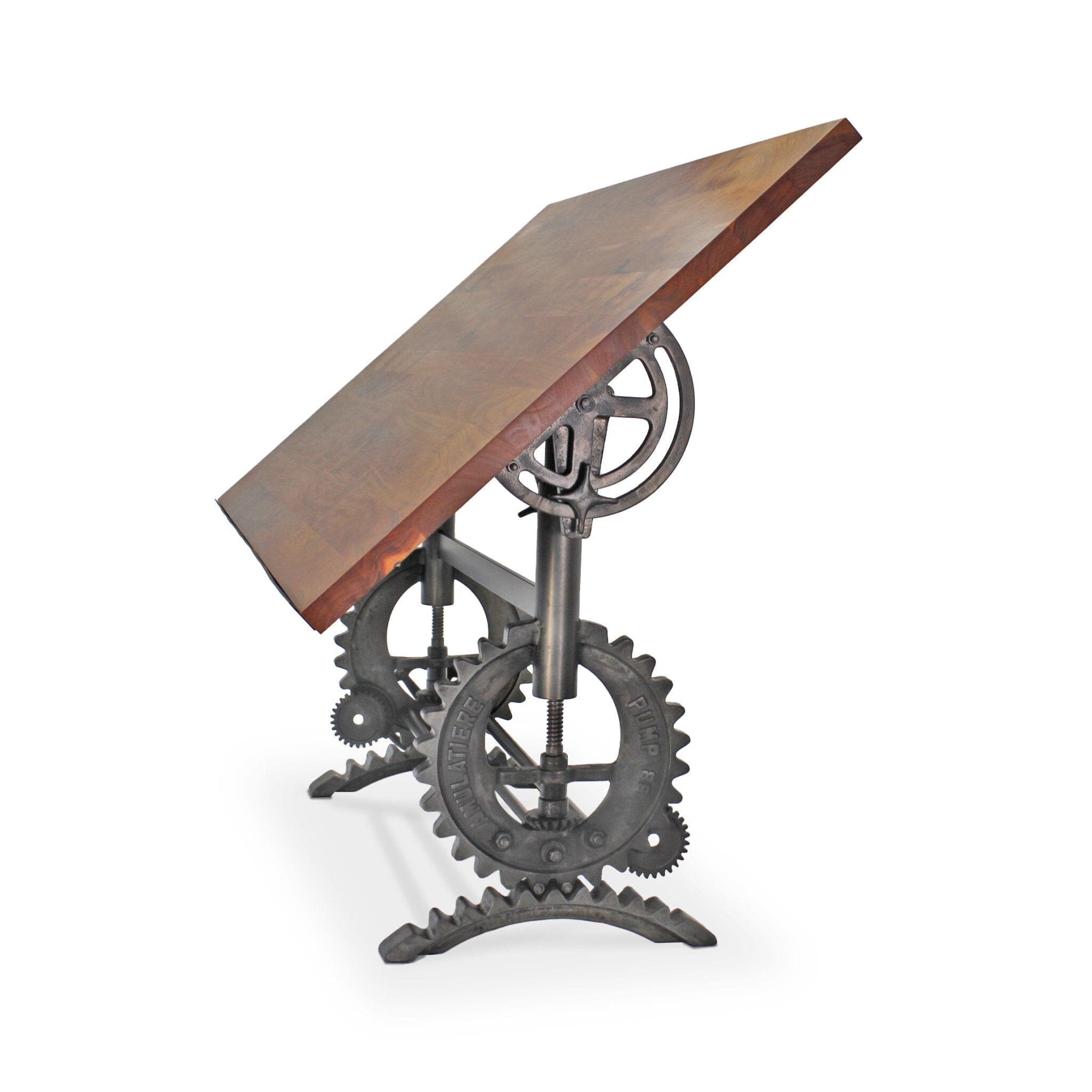The image showcases a detailed drawing of an old-fashioned drafting table. The centerpiece of this machine is a large, sturdy wooden tabletop, likely crafted from mahogany, that rests diagonally over an intricate metallic base. The brown tabletop, measuring approximately four feet by four feet, is supported by an elaborate system of interconnected gears and cogs of varying sizes, which provide the functionality to tilt the table at different angles. These gears are complemented by circular and straight metallic rods forming the structural support. Beneath the table, there are two wheels on the floor, with arc-shaped feet supporting them, adding to the table's adjustability. The entire setup is set against a clean, white background, highlighting the mechanical complexity and vintage charm of the drafting table.